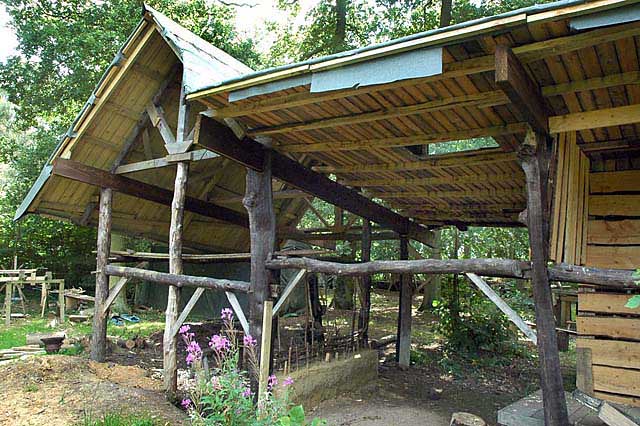The image captures a rustic, wooden structure, possibly a home or barn, situated outdoors in what appears to be a forested area. The building is constructed from uneven wooden planks that have gaps between them, contributing to its rough-hewn charm. The roof, made entirely of wood, is held up by thick, uncut logs that retain their natural form. This main structure features a square hole in the center of the breezeway and a shaded garden area covered by an angled roof. Surrounding the building is a tree limb fence, along with a rock walkway that meanders through a grassy area punctuated with patches of bare ground. Vivid purple and pink flowers are in bloom near the tree trunks that serve as support poles for the structure. In the background, lush trees complete the serene, nature-rich setting, indicative of an outdoor scene taken in the middle of the day. The color palette of the image includes shades of light brown, green, gray, pink, and dark brown. There is no text present in the image.